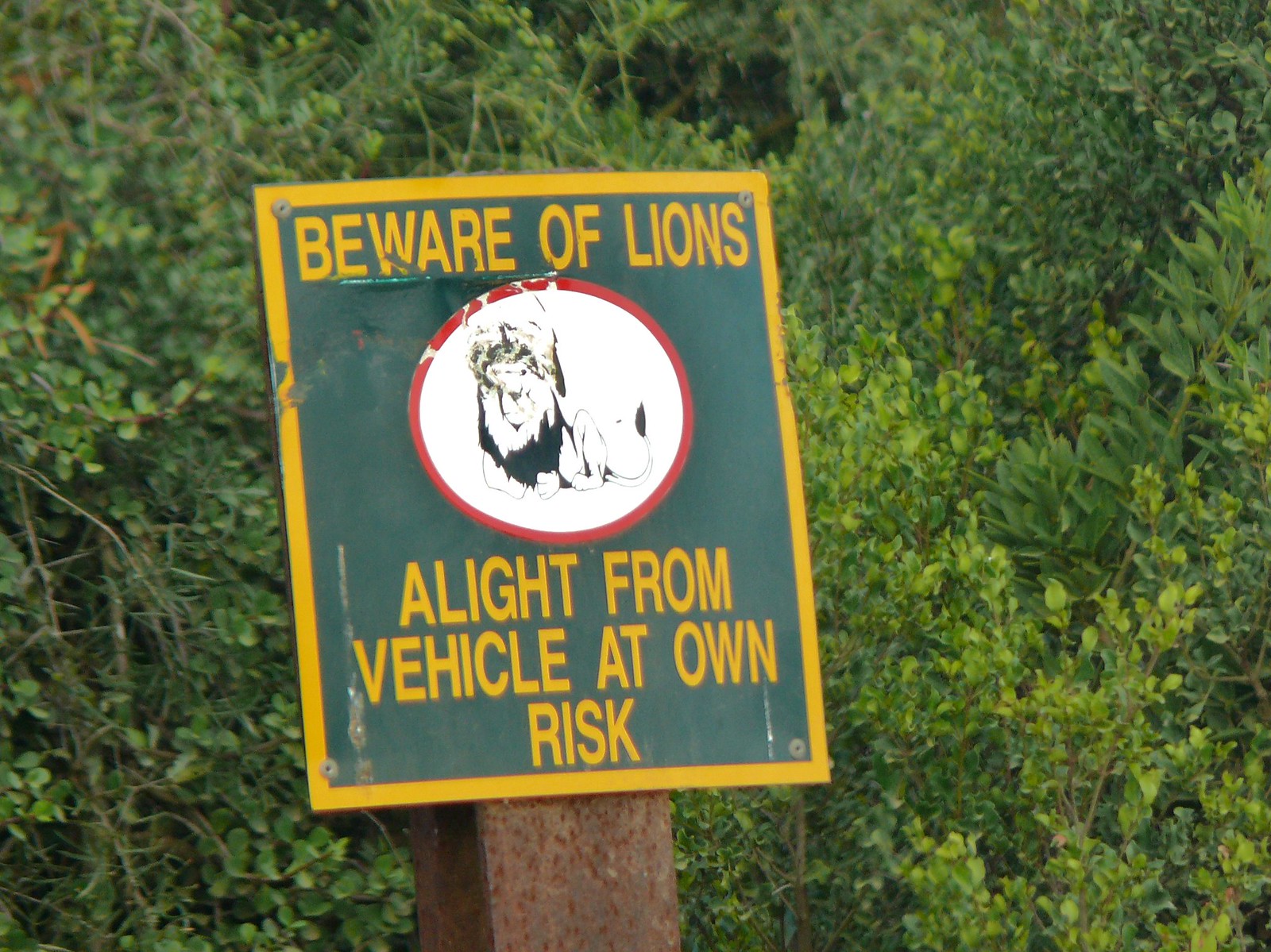In the center of the image, a weathered metal sign is mounted on a thick, rusty pole. The sign has a yellow border with sections that appear to be worn and scratched. The main part of the sign is gray, with bold yellow text at the top that reads "BEWARE OF LIONS." Below this, a white circle with a red border features a somewhat cartoony black-and-white lion icon. Beneath the circle, more yellow text warns, "A LIGHT FROM VEHICLE AT OWN RISK." The background is filled with dense greenery, predominantly a mix of trees and bushes, indicating an outdoor setting in what seems to be a dangerous, wilderness area. The image captures the vivid greens and various shades of brown and yellow, along with some traces of dark blue, likely from shadows or the play of light. The scene suggests it is taken in the middle of the day, emphasizing the stark contrast between the sign and its lush surroundings.